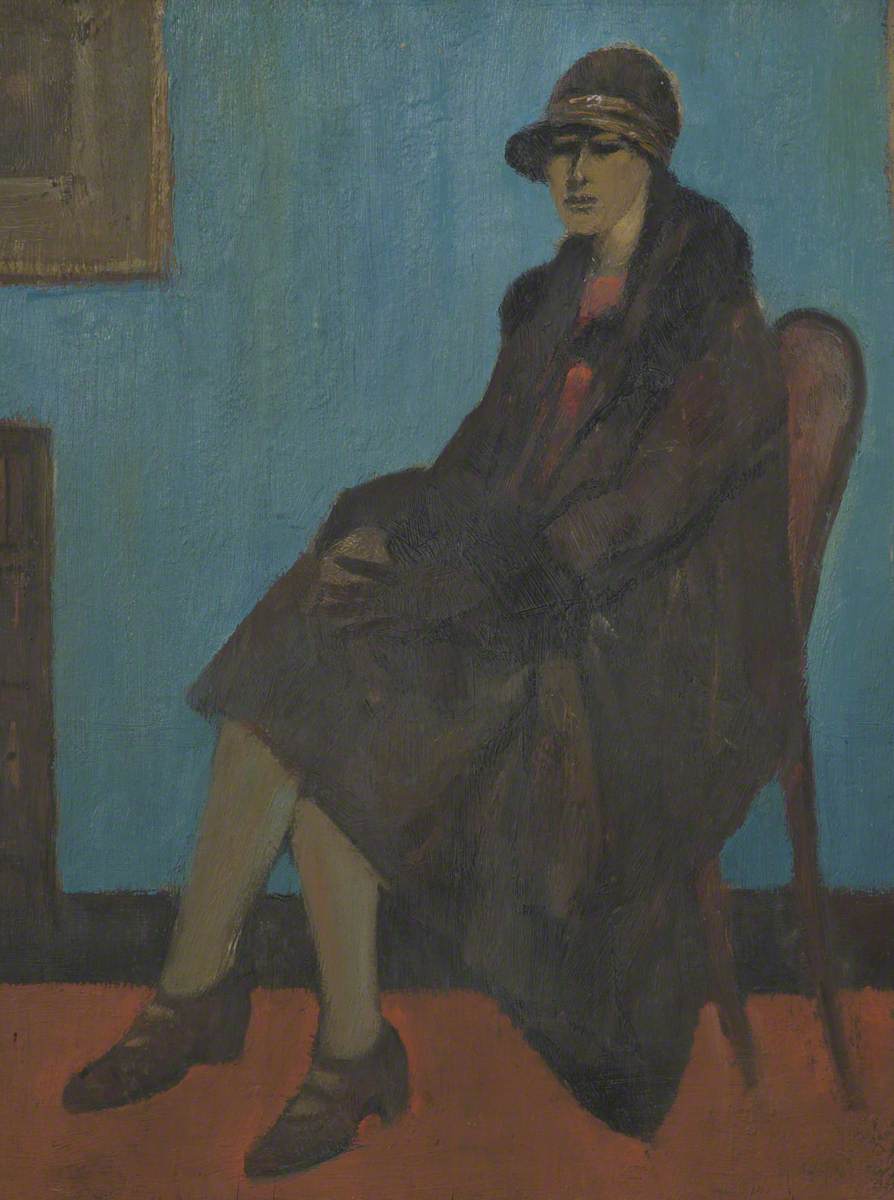This vertical rectangular painting depicts a woman seated in a brown, straight-backed wooden chair indoors, in a room with a dark blue wall. The woman, seemingly an heir of the flapper era, has a somber expression and is clad in muted tones. She wears a dark brown cloche hat with brims down, a brown coat that hangs open over the chair, partially revealing a colored dress underneath. Her ashy complexion is detailed with long features and dark eye sockets, though the painting's style blurs these details into a muted blend. Her legs, clad in grayish stockings, are crossed and she wears dark brown heeled Mary Jane shoes. Her gloved hands rest in her lap. The background highlights the blue wall with a trim of dark wood at the bottom. A framed picture, only partially visible, and the corner of another household item, possibly a dresser, can be seen. The floor is a reddish-brown hue, adding a touch of warmth to the otherwise muted scene.